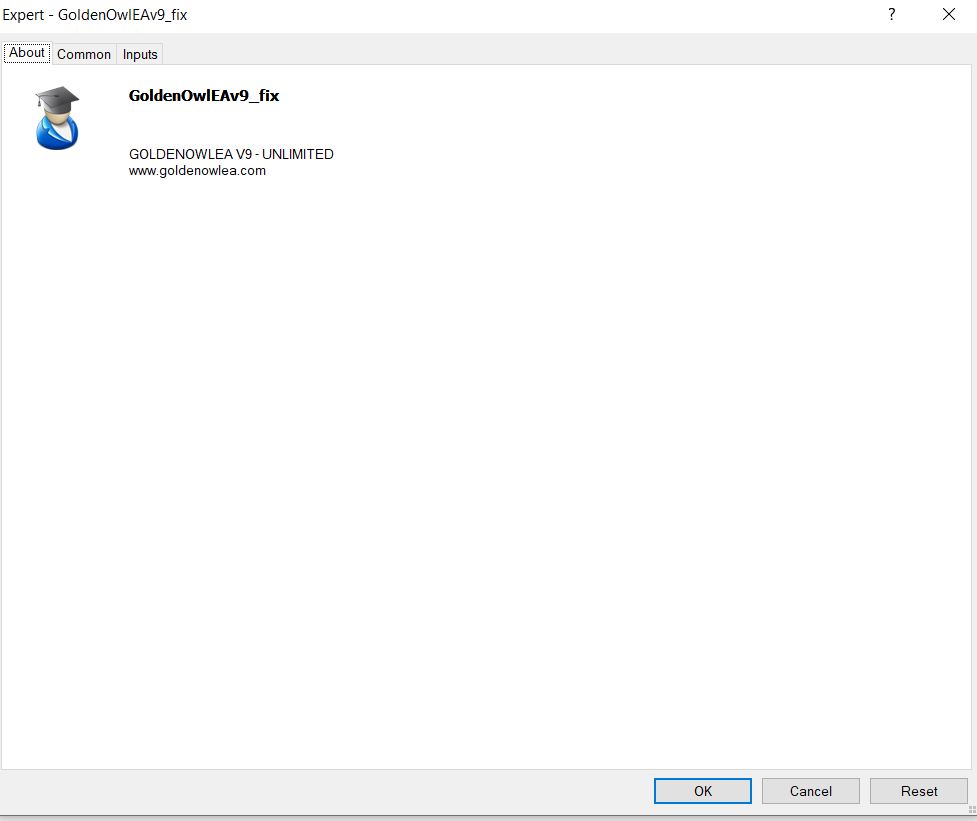A highly specialized interface shows the detailed setup process for the "Golden Owl EAV9" expert advisor. The interface includes multiple options such as "OK," "Cancel," and "Reset" for managing common inputs. The version displayed is "Golden Owl EAV9_Fix" with an "Unlimited" usage model. For more detailed information, the official website www.GoldenOwlEA.com is provided at several points on the screen.